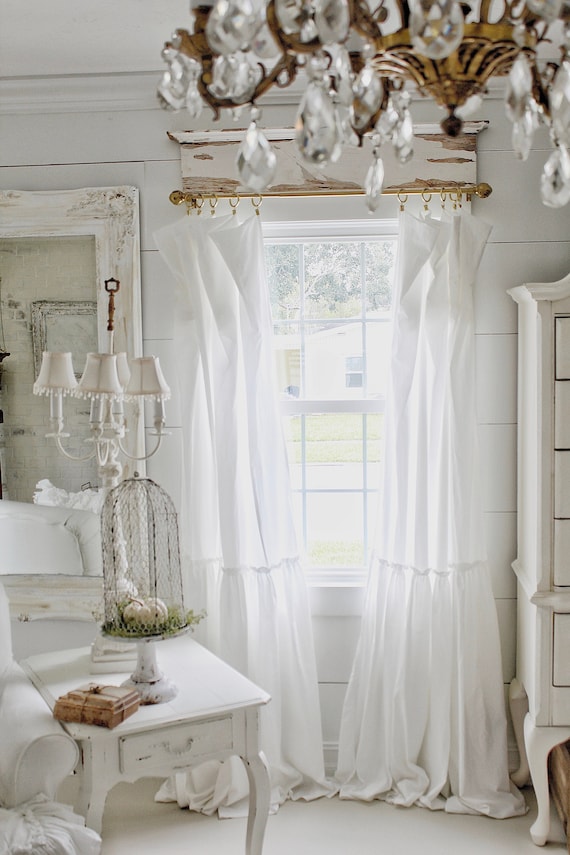This photo captures a romantic, rustic-themed bedroom corner, showcasing an elegant and serene atmosphere. Dominating the center of the white shiplap ceiling is a gold chandelier adorned with crystal egg-shaped lights, casting a romantic glow. Directly in front of us, a large window is dressed with flowing white curtains hanging from a gold rod. 

To the right of the window stands a classic five-drawer chest with distinct Queen Anne-style legs ending in clawed feet, maintaining the room's white color scheme. A single-drawer table sits to the left, topped with a brown gift box and a decorative item resembling a small cage. Next to the table is a cozy white armchair, while a reflective large rustic mirror echoes the room's romantic allure.

In the background, a bed is partially visible, tucked away but contributing to the room's cozy intimacy. A white-based three-lamp stand with white shades further illuminates the space, ensuring every corner of the room is bathed in a soft, inviting light.